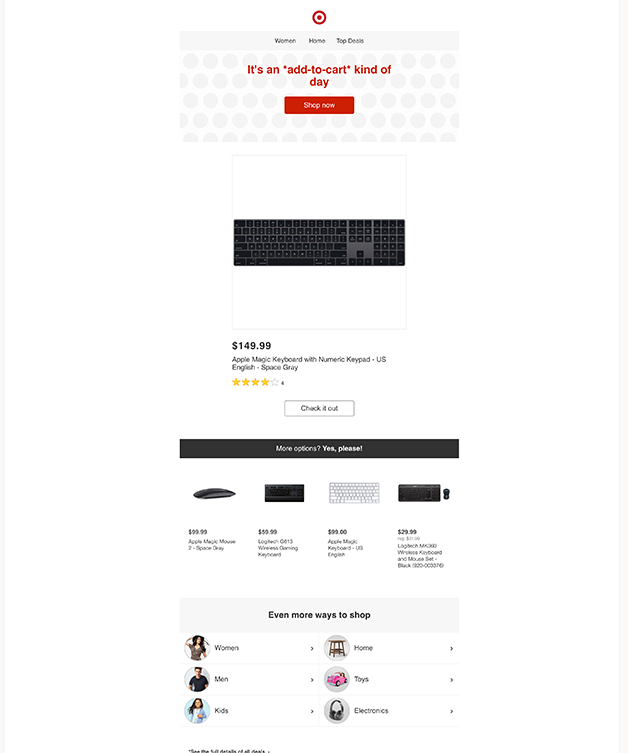A screenshot from a mobile phone displays the Target website. The top part of the screen shows the Target branding and a navigation breadcrumb reading "Women > Home > Trip Details." The background has a white hue with light gray circular patterns resembling wallpaper. Prominently featured in red text is the phrase "It's an add to cart kind of day," accompanied by a red "Shop Now" button with white lettering.

Below this button, there's a listing for a keyboard priced at $149. The product has a four-star review rating, and there is a "Check it out" link available for more details. Following this, four different keyboard options are presented with brief descriptions.

At the bottom, there's a section titled "Even more ways to shop," which includes clickable links for various categories: Women, Men, Kids, Home, Toys, and Electronics. The overall layout is user-friendly with intuitive navigation options to explore products further.